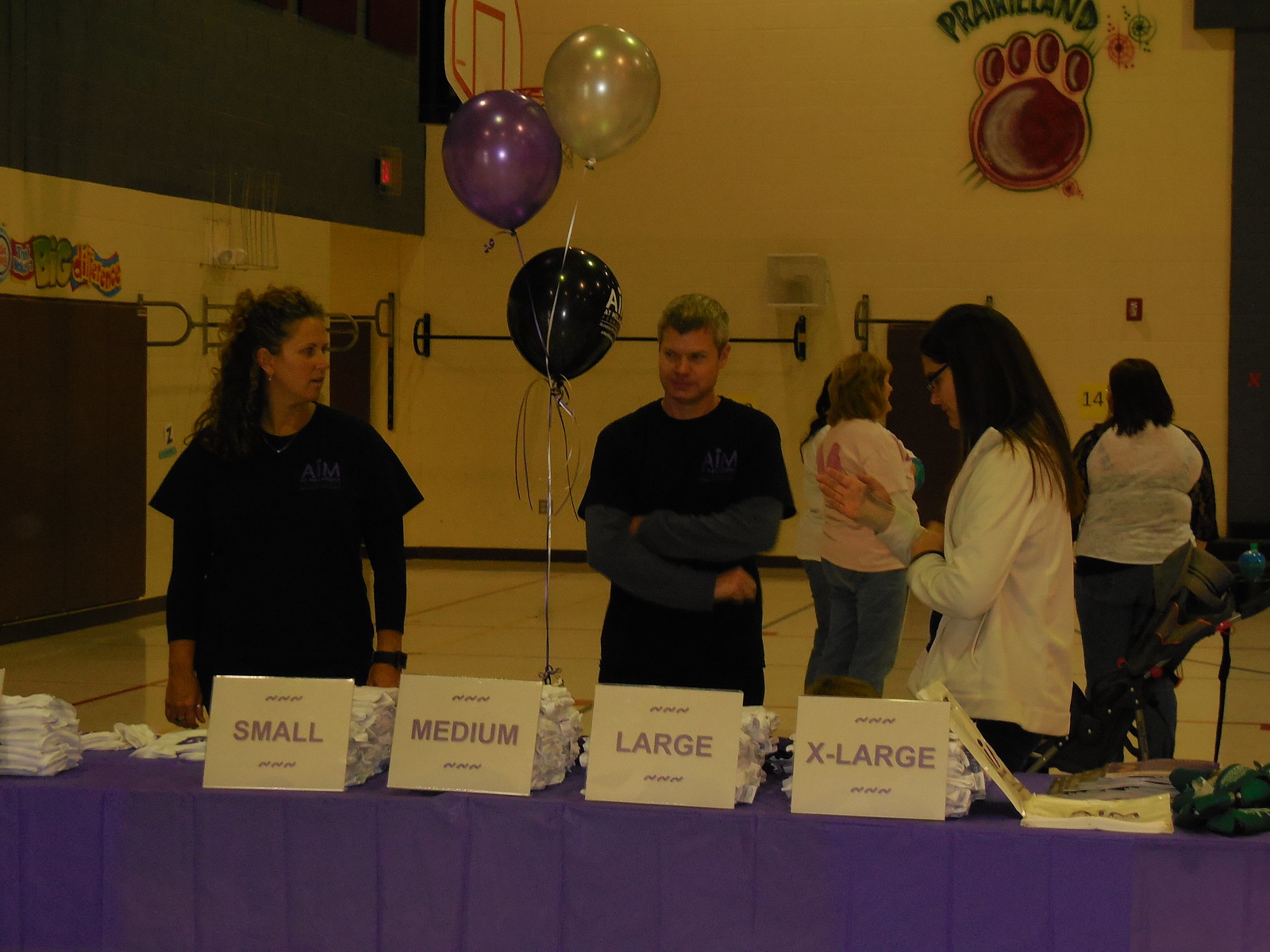This detailed photograph, taken inside what appears to be a school gymnasium with dim lighting, captures a busy scene anchored by a prominent table covered in a purple cloth. On the table, there are four neat stacks of T-shirts, each labeled with sizes—small, medium, large, and extra-large. The labels are clearly marked on pieces of paper placed in front of each stack. Attached to the table are balloons in gold, purple, and green, adding a festive touch to the setting. 

Behind the table, five people are standing: a woman on the left, a man in the middle, and another woman to his right, flanked by two more women further back. All individuals appear to be wearing school uniforms, possibly indicating a school event or sale. The gymnasium's walls are yellow, and notable in the background is a graffiti-style paw print, hinting at the school's mascot or team. There also appears to be gym equipment such as pull-up bars and an emergency exit door in view, alongside an indistinct catchphrase or slogan painted on the wall.